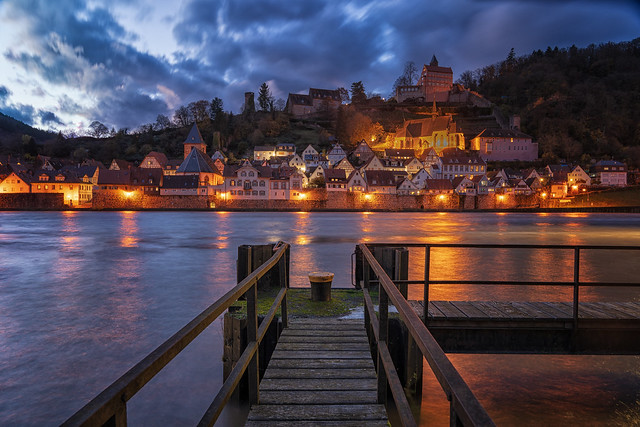The image captures a picturesque, nighttime scene of a quaint European village nestled on the edge of a serene body of water, possibly a lake or calm river. The foreground prominently features a wooden dock, painted in various shades of brown, extending from the bottom and veering to the right, hovering above the still, reflective water. This water mirrors the village's softly glowing amber lights, creating an enchanting, almost magical ambiance.

The village itself showcases a collection of white homes with brown, triangular roofs, perched both along the shoreline and ascending the gentle slope of a hill. The houses exude a charming, chalet-style aesthetic typical of European cottages. Nestled amongst these homes are small, dark green trees, adding to the serene, natural beauty of the scene. A hint of a green moss with a bucket atop is visible near the dock, providing a touch of rustic authenticity.

In the background, gentle curved hills rise with dense clusters of very dark, foresty green trees, blending into the dusky, deep blue sky. The sky itself, heavy and overcast with clouds, suggests an approaching nightfall, contributing to the overall dreamy and tranquil atmosphere of the setting.